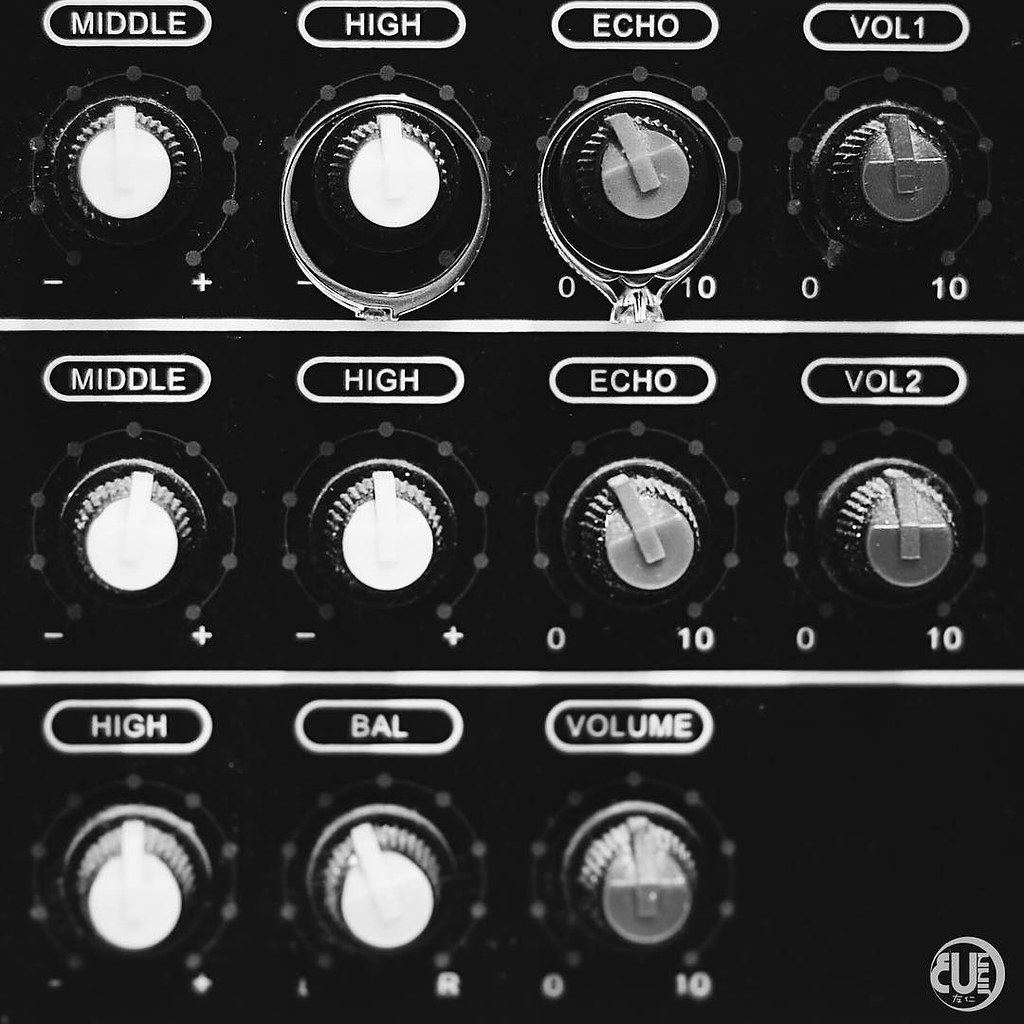This black and white photograph captures a close-up view of an audio equalizer panel with 11 meticulously detailed knobs arranged in three rows. The top row houses four knobs labeled, from left to right, as middle, high, echo, and volume 1 (VOL 1). The middle row mirrors this setup with another set of middle, high, echo, and volume 2 (VOL 2) knobs. The bottom row contains three knobs labeled high, balance (BAL), and volume. Each knob features various indicators and symbols, including minus and plus signs for adjustment, numerical scales ranging from 0 to 10, and some with L (left) and R (right) designations. Above each knob is a long oval-shaped area, providing a clear space for labeling. The color distinction under the knobs includes white and gray shades, aiding in differentiating control functions. This image, with its heavy use of Photoshop to emphasize the monochrome effect, showcases the intricate design and precision required for audio engineering.